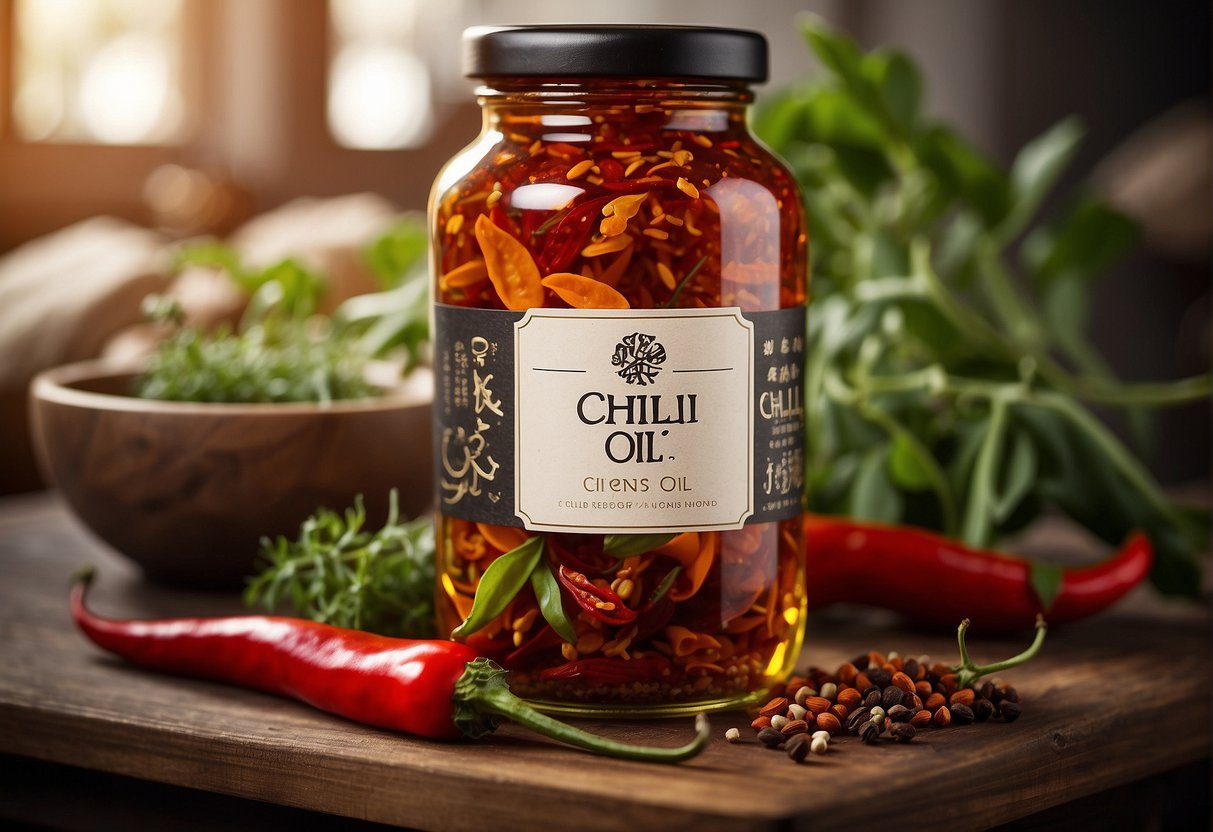The high-quality culinary photograph, likely suited for a cookbook or culinary magazine, is staged on a wooden tabletop in landscape orientation. The background, intentionally out of focus, suggests the setting is a kitchen. Dominating the center of the image is a clear glass jar with a black screw-on lid, visibly filled with a light amber chili oil packed with dried chilies, toasted dried garlic, and possibly sesame seeds. The jar's label, although marred by apparent AI-generated artifacts, reads "CHILI OIL" with a peculiar rendering of the letters "I-I" in "CHILI."

To the left side of the table, a handcrafted wooden bowl holds an assortment of fresh herbs, while directly to the right lies a fresh herb with large green leaves, partially cut and casually placed on its side. Two vibrant red chili peppers are artistically arranged on the table, one pointing right with its stem, the other in the opposite direction. Scattered on the wooden surface next to them is a colorful pile of peppercorns, including white Sichuan peppercorns, red, and black varieties, alongside possible coriander seeds.

This intricately composed photograph emphasizes the jar of chili oil as the focal point, showcasing its rich content and exotic appeal against a backdrop of complementary culinary ingredients.